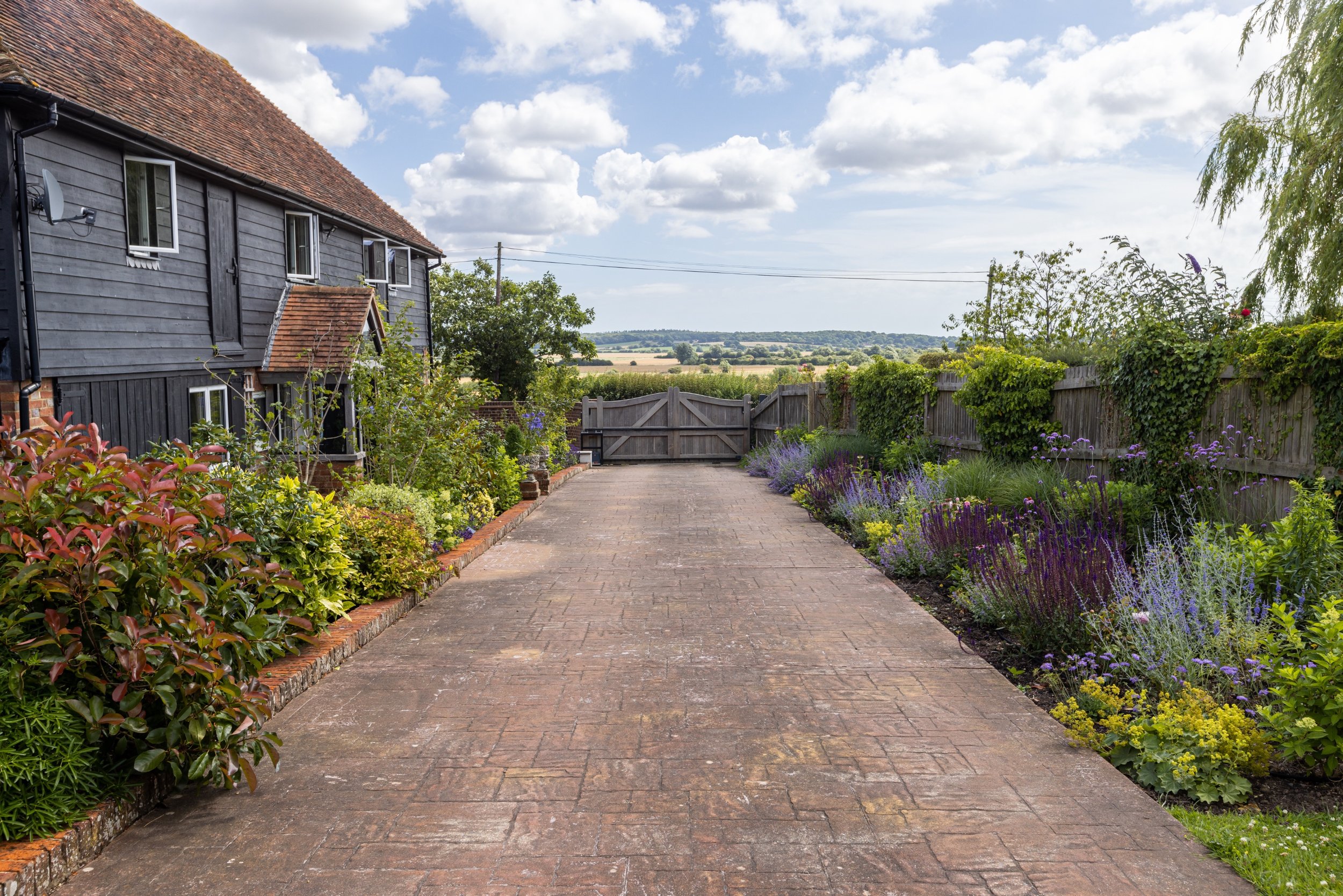The image captures a scenic outdoor setting under a blue sky dotted with white and gray clouds. Dominating the left side of the image is a gray, two-story house with white-framed windows and a satellite dish attached to its side. This building is topped with a brown rooftop and appears to be somewhat aged. Surrounding the house is a gray fence, and just beyond it lies a green, field-like expanse with shrubs and trees.

In the foreground, a well-maintained garden flourishes with an array of colorful flowers. Predominantly on the right side, the garden has clusters of purple and yellow flowers, with additional shrubs lining both sides. The garden's pathways are adorned with landscaping materials, and the ground itself appears to be made of brown stone, creating a clear separation between different sections of the garden. 

Power lines on poles stretch across the image, hinting at the presence of modern amenities despite the rustic charm. The sun shines brightly over the scene, illuminating the meticulously cared-for plants. A brick driveway or sidewalk runs through the foreground, leading to a gate that seemingly allows vehicle access to the property. In the distance, a mountain range serves as a majestic backdrop to this tranquil and picturesque setting.